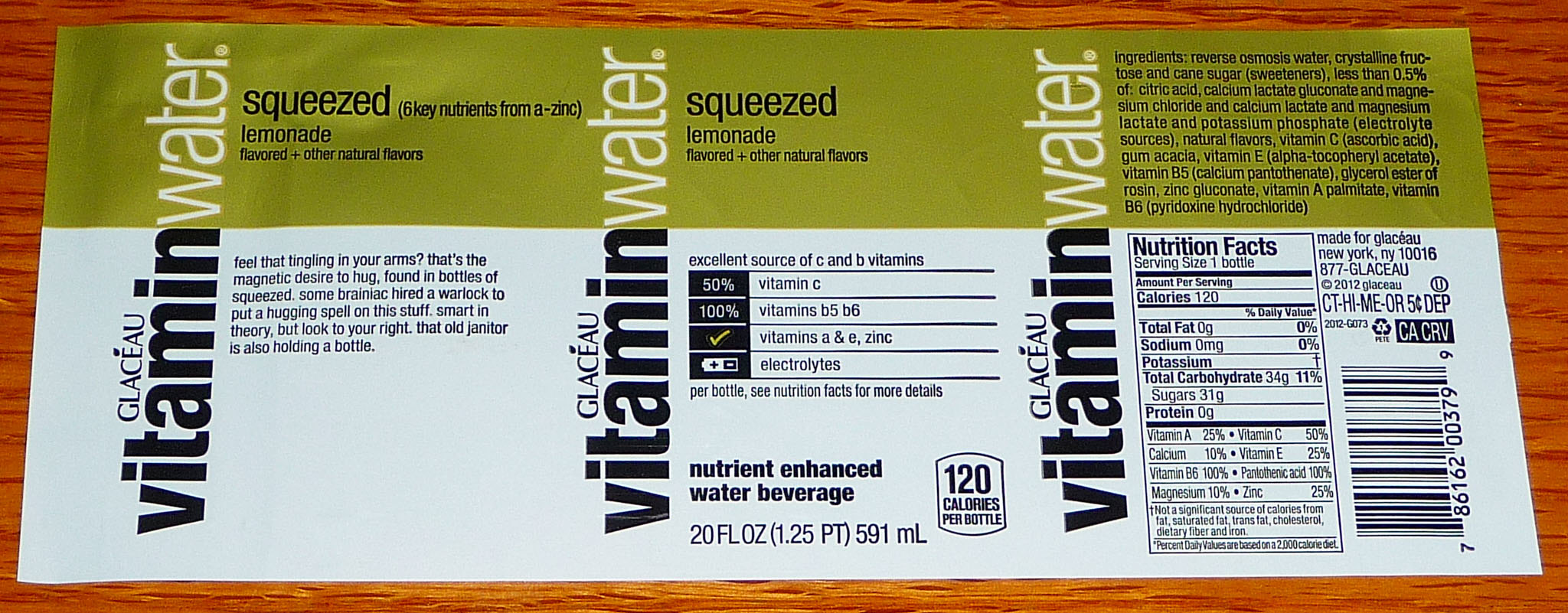This detailed image features an elongated and narrow label from a Glacéau Vitamin Water bottle, specifically of the "Squeezed Lemonade" flavor with additional natural flavors. The label is at least three times as wide as it is tall, and is sectioned into three distinct panels.

The first panel, located on the left, highlights the benefits and suggested uses of the beverage. The second, central panel, lists the enhanced nutritional values, detailing the various vitamins and electrolytes that the drink contains. The third panel, positioned on the right, provides comprehensive nutritional facts, the targeted consumer group, and an ingredient list positioned above this information.

Visually, the label’s top third is distinguished by its vibrant lemon-green color. The word "Water" from the product’s title is prominently displayed in white, while "Squeezed" is written twice in bold black lettering. The ingredients are also printed in black within this section. Meanwhile, the lower two-thirds of the label serves as a contrasting white background with all text rendered in black, ensuring clarity and readability for the informative content displayed.